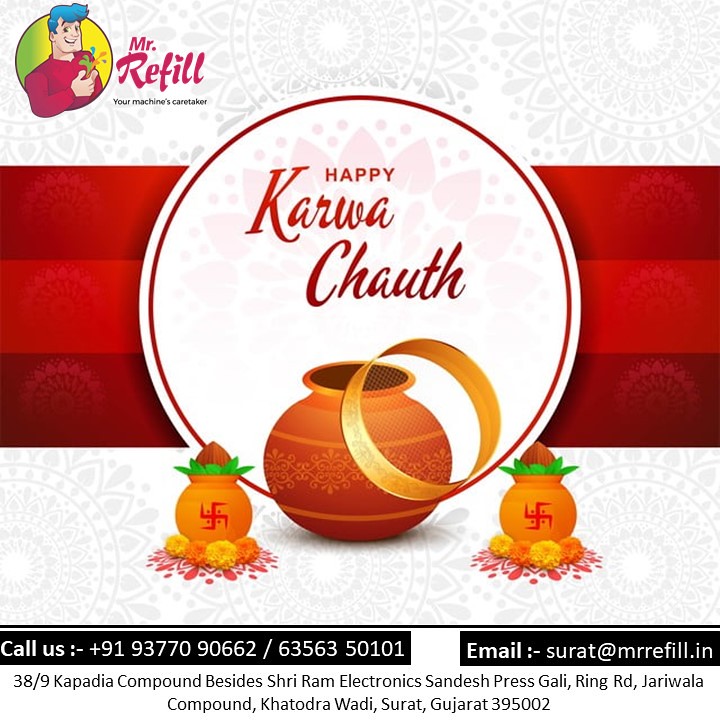The advertisement, set against an off-white background adorned with light gray sunflowers featuring Oriental-style designs and dots, prominently displays the branding for Mr. Refill, "your machine's caretaker." In the upper left corner, the Mr. Refill logo includes a whimsical cartoon man with blue hair, wearing a pink shirt, with splashes of colors emanating from his hands, next to pink text stating "Mr. Refill." Central to the design are three horizontal red stripes—dark red on the top and bottom, bright red in the middle—overlaid with a bold white circle framed in red. This circle contains the red text "Happy Karwat Kuff." Below this, a gold ring leans against an orange pot that features gold trim and intricate designs. Additionally, there are smaller pots embellished with red swastikas and green, leafy plants at the bottom of the image. The advertisement provides contact information: call +91-93770-90662/63563-50101, email surat@mrrefill.in, and the address, 38/9 Kapita Compound, beside Shree Ram Electronics, Sandish Press Gali, Ring Road, Jawala Compound, Kahudrawadi, Surat, Gujarat 395002.